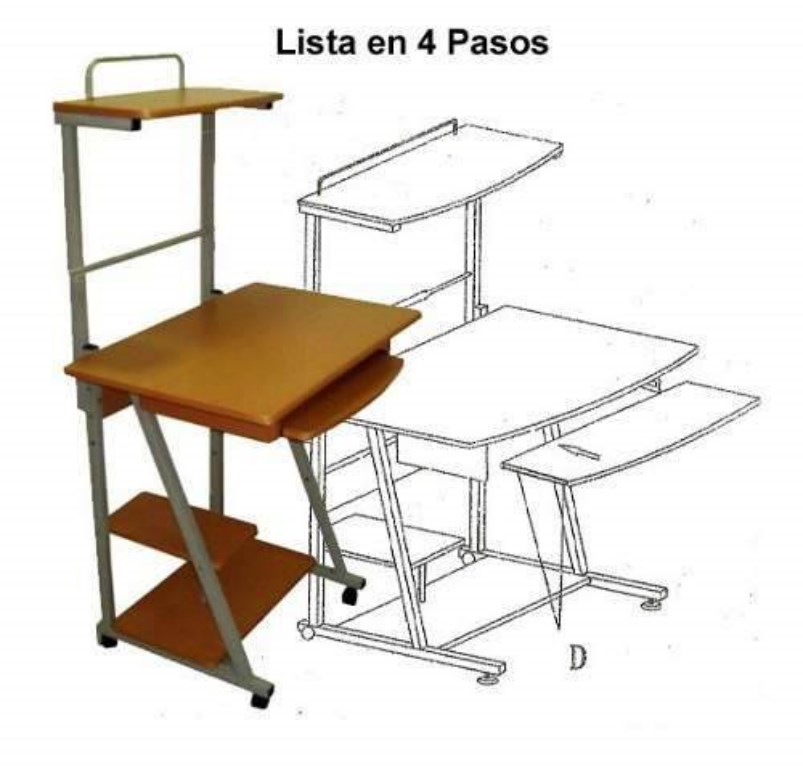The image depicts a portable desk made of tan wood with a sturdy metal frame. It features multiple shelves and storage compartments, including a large wooden desktop, a pull-out keyboard tray, and several side shelves of varying sizes. The desk is equipped with wheels, allowing it to be easily relocated, and has a handle on top for convenient maneuvering. The left side of the image shows the actual desk, while the right side displays a black and white line drawing of the same desk, illustrating its design and components. The illustration includes text at the top, which reads "Lista N4 Pesos," and a handwritten letter "D" in the bottom right corner. The detailed diagram highlights the desk’s functionality and compact design, emphasizing its practicality for versatile use.